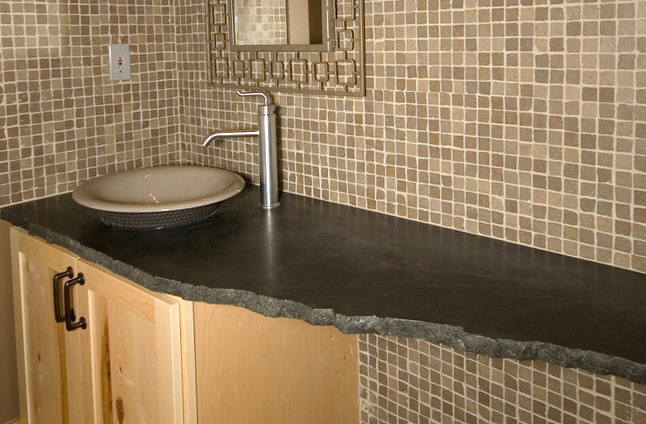This image showcases a meticulously designed bathroom area. At the center is a distinctive countertop made of green granite with a jagged, rough edge, adding a touch of natural elegance. Atop the countertop sits a bowl-style sink, positioned above the surface for a stylish, modern look. The sink is paired with a sleek, silver single-handle faucet.

In the background, the wall is adorned with small brown mosaic tiles, offering a textured, intricate backdrop that complements the countertop's rough edges. The cabinets beneath the granite countertop are crafted from light wood, possibly blonde oak or maple, adding warmth and brightness to the overall aesthetic.

Above the countertop, a unique mirror blends seamlessly with the mosaic tile. The mirror's frame appears to be made of metal with open sections that align perfectly with the tiles behind it, creating an integrated and harmonious design. Additionally, a silver light switch is mounted on the wall, subtly embedded into the backdrop without disrupting the cohesive design.

The entire composition of the bathroom area speaks to a sophisticated blend of natural materials and modern design elements, resulting in a serene and inviting space.